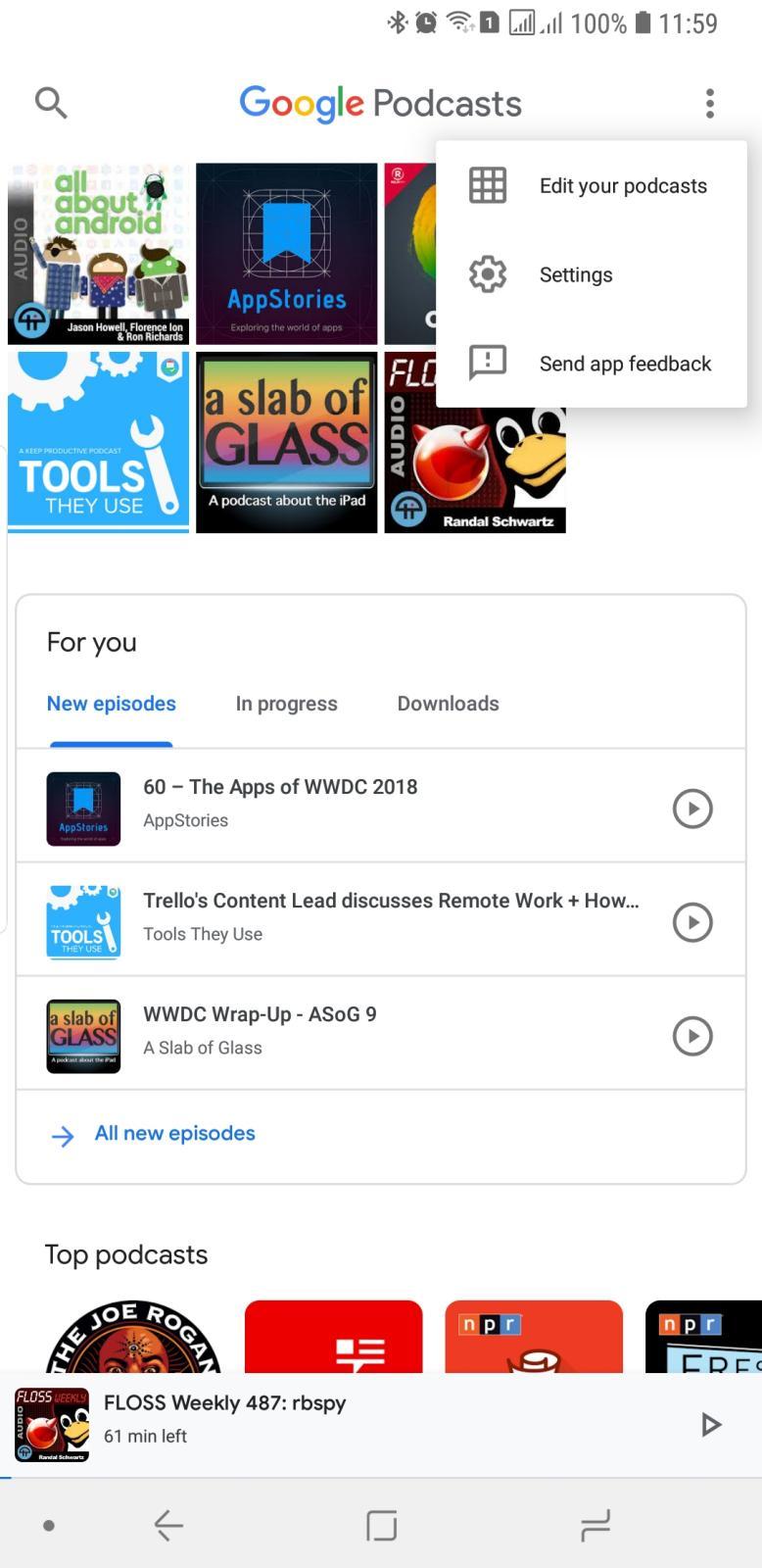In the image, which appears to be a screenshot from a smartphone, the status bar at the top right corner displays a Wi-Fi icon, a fully charged battery at 100%, and a time of 11:59. On the top left, there's a search icon. Centrally located at the top is the title "Google Podcasts."

A pop-up menu on the right side of the screen presents three options: "Edit your podcasts" (accompanied by a grid icon), "Settings" (featuring a gear icon), and "Send app feedback" (with an exclamation mark icon). 

Behind this pop-up, the main screen is visible, showing six podcast thumbnails. The first podcast titled "All About Android" displays an image of three robots. Another podcast appears to be titled "App Stories." The third podcast is partially obscured by the pop-up menu. The fourth podcast, labeled "Tools," features imagery of various tools and gears. The fifth shows a slab of glass, and the sixth has an illustration of a bird.

Beneath these thumbnails, a horizontal menu labeled "For You" includes tabs for "New Episodes," "In Progress," and "Downloads." The "New Episodes" tab is highlighted in blue and underlined. The three episodes listed under "New Episodes" are titled: "The Apps of WWDC 2018," "Trello's Content-Led Discussion on Remote Work," and "WWDC Wrap-Up ASOG 9."